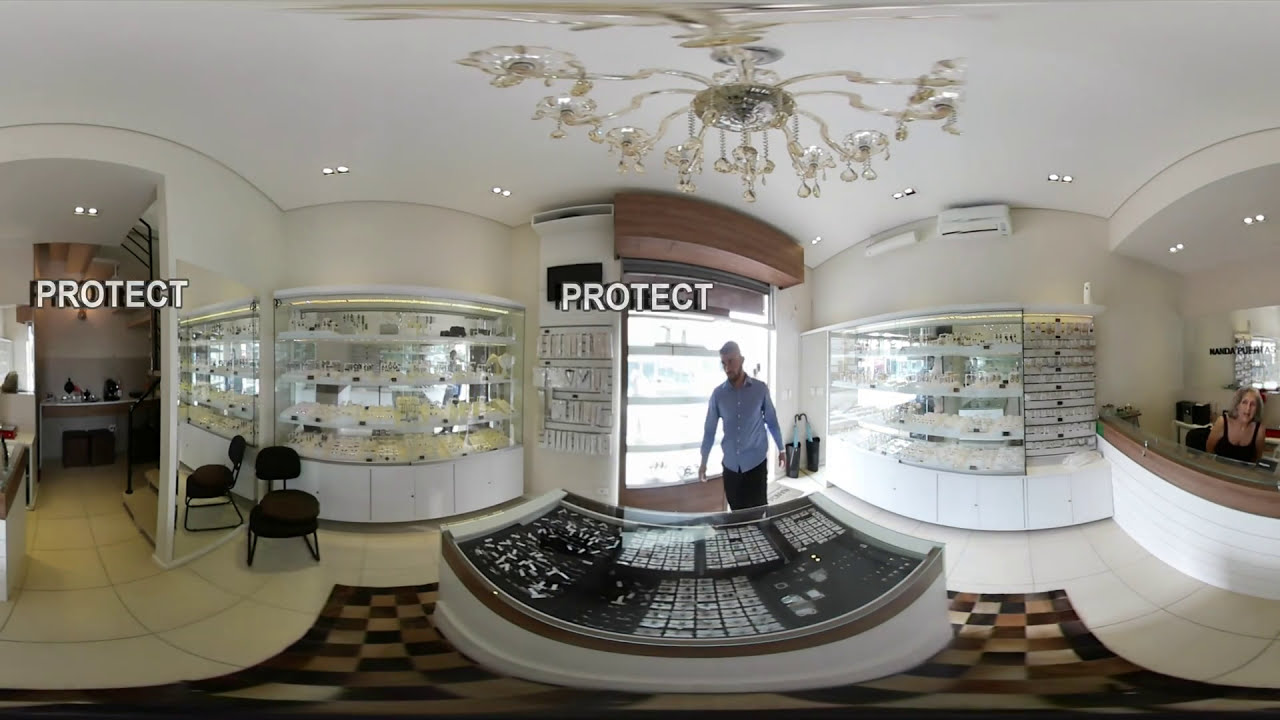The image depicts the interior of a jewelry store, likely captured by a camera, which appears slightly distorted. The scene features a man in the center, donning a blue button-up shirt with a collar, dark pants, and glasses. He walks on a checkered carpet composed of dark brown, light brown, tan, and beige squares, transitioning to a white tile floor on the right. The main focal point is a large, rectangular jewelry display case in the center, which appears warped at the ends. This case, adorned with numerous white squares likely housing jewelry, such as necklaces or rings, sits atop a checkerboard-patterned floor. 

In the background, the walls curve outwards, each featuring four shelves above large cabinet doors. Overhead, a grand chandelier illuminates the scene. The word "PROTECT" overlays the image twice in white font with a black shadow—once on the left edge and again in the center, beneath the chandelier. 

To the right, there's a girl in a black dress seated behind a counter, while to the left of the central display, there are chairs positioned in front of additional glass cases. The predominant color scheme is a clean white, extending from the floors to the ceiling, contributing to the elegant and secure atmosphere of the store.